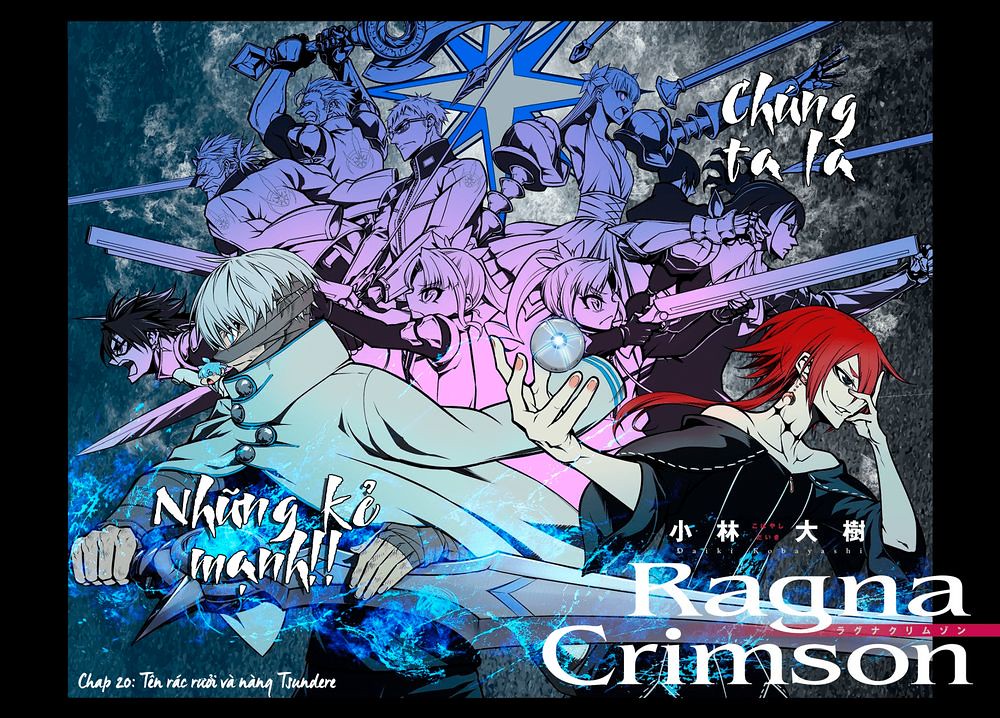This compelling image appears to be a scene from a manga or graphic novel titled "Ragna Crimson." The visually dynamic composition is dominated by bluish and purplish hues, creating a monochromatic background where anime characters are depicted in combat stances. These characters, armed with guns and swords, are arranged in a circular formation, suggesting a united front against an impending challenge. Their figures fade in intensity towards the background, culminating in a subtle blue star that pierces the distant sky.

In the forefront of the scene are two striking main characters. On the left stands a male figure, possibly named Nyung Kae Mon, clad in a Victorian-style cape adorned with large buttons and a face wrapped in gray bandages. His spiky white hair contrasts with the blue energy emanating from the large sword he wields, and his gaze is directed to the left. To the right is a woman in a black sorcerer's robe with short red hair. She holds a floating metal orb between her fingertips, her other hand raised to her face in a gesture that hints at a forthcoming attack, her sly smile brimming with confidence.

The image is accented with various textual elements. At the top right, the phrase "Chung to La" is displayed in an Asian script, while "Ragna Crimson" is prominently featured in bold letters at the bottom. The bottom left corner includes additional Asian text alongside "Chapter 20;" although some wording remains illegible, these details contribute to the rich, immersive narrative quality of the image.